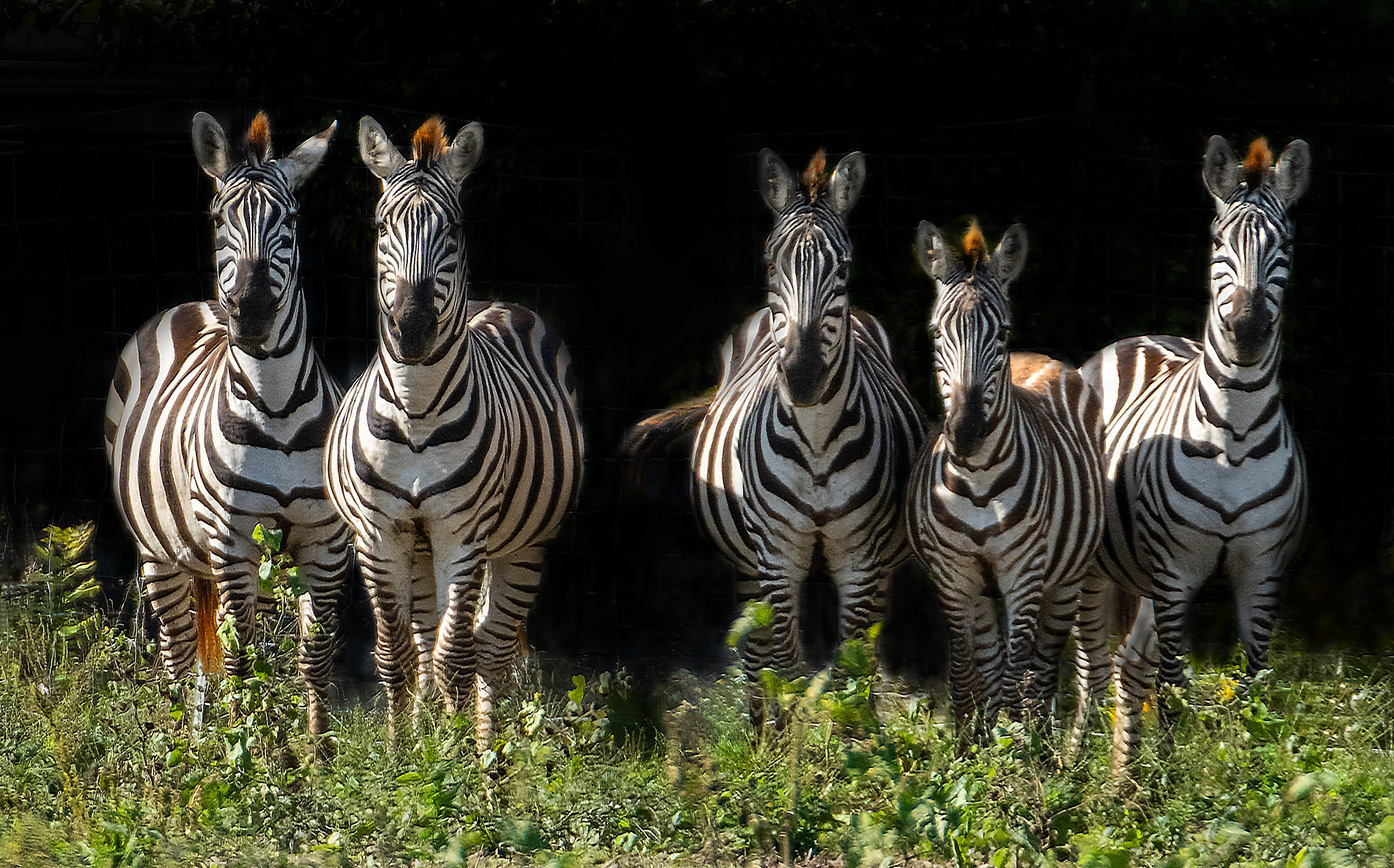This photo captures a group of five zebras standing in a lush, grassy field with tall stalks of green and hints of yellow reaching up to their bellies. The zebras, with their iconic black and white stripes, stand at attention, fixated on the photographer, suggesting they are intrigued or engaged by the person behind the camera. There are two zebras on the left and three on the right, separated by a small gap. Beyond them, the background is almost entirely black, suggesting potential digital or AI alterations. Each zebra has a peculiar addition—a small, orange tuft resembling a candle wick with a flame on top of its head. The overall scene is surreal due to this unusual feature and the darkened backdrop, giving it an otherworldly ambiance.